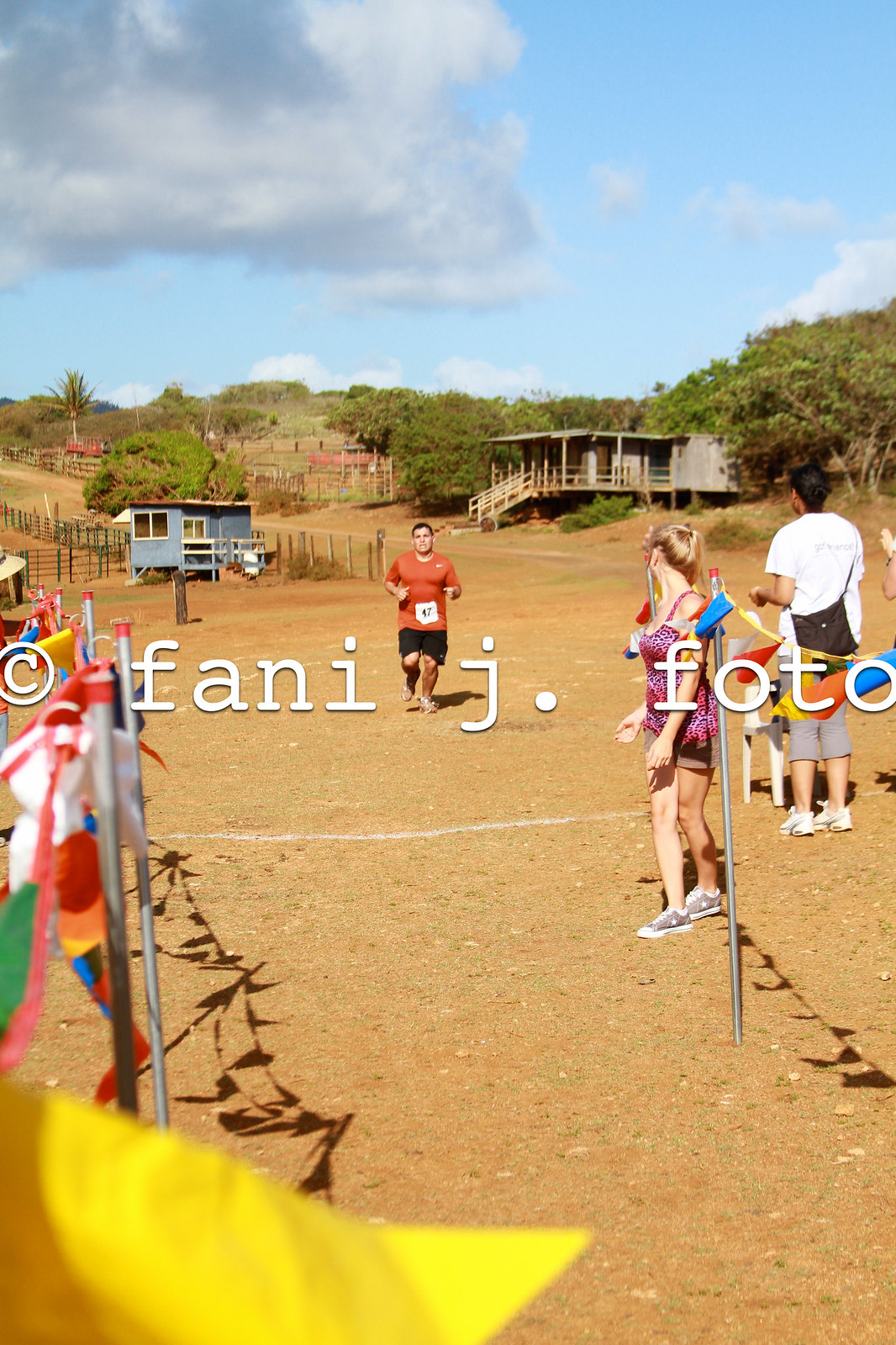In this picturesque outdoor scene, captured by fannyj.photo, a thrilling race reaches its climax as a man in a red shirt and black shorts, wearing race number 47, sprints towards the finish line. The dirt road underfoot winds through an open rural area, with green hills and scenic tree lines in the background under a vivid blue sky dotted with a mix of white and grayish clouds. The finish line is marked by multicolored flags strung between five-foot metal poles and a white chalk outline on the ground.

Spectators are scattered along the sides of the road, cheering on the racers. On the right side, a woman in a purple spaghetti strap shirt and black shorts appears to shout encouragement to the approaching runner, her back turned to the viewer. Nearby, another lady dressed in a white t-shirt and gray capri pants, with dark hair tied in a bun and a brown sling bag, also watches the competitors with excitement. A third person, partially visible, is clapping enthusiastically.

In the background, two wooden structures can be seen— a small blue house on the left and a larger gray house on stilts to the right— adding to the rural charm of the scene. This photo captures not just the intensity of the race but also the communal spirit and rustic beauty of the location.